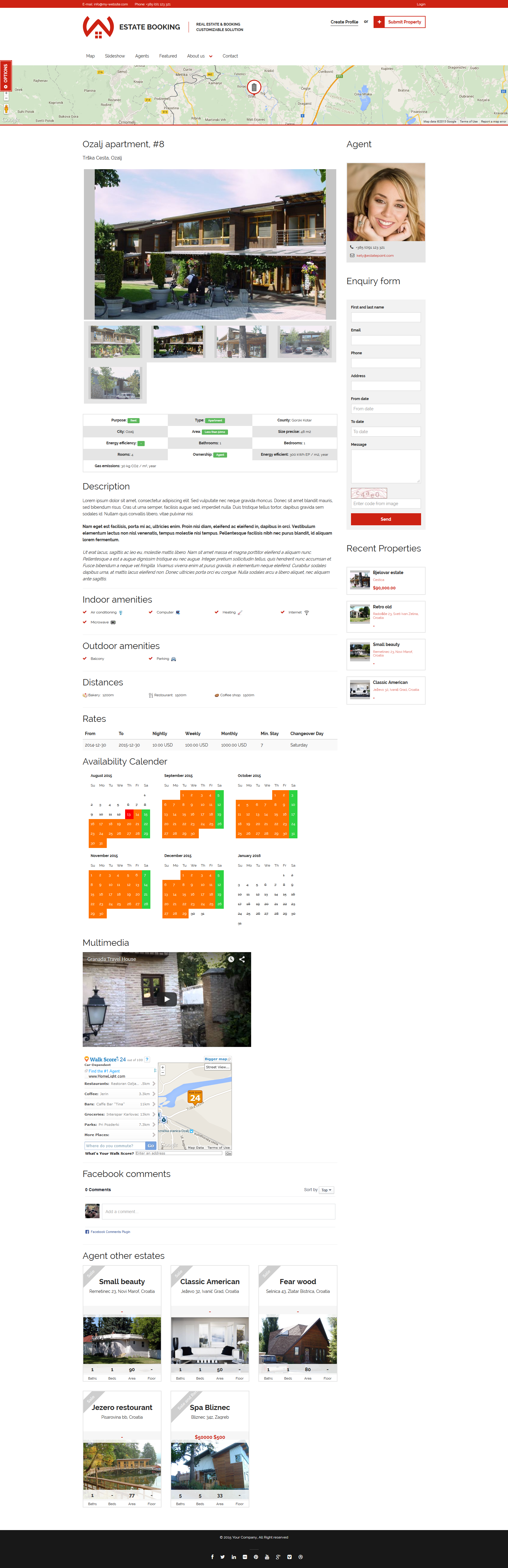The image depicts a detailed real estate webpage featuring a prominent picture of a female agent labeled "Agent" above her name. In the background, there is an image of a multi-unit apartment building. The webpage includes small-font text, presumably descriptions of the various apartment units, which are difficult to read. At the top of the page, the header reads "Estate Booking" accompanied by an orange or red logo resembling the letter "W" with a unique design. Below the agent’s photo, there are fields for visitors to input their name, email, and contact information. Further down the page, an availability calendar is visible, showing different available dates for potential bookings. Overall, the webpage appears to be designed for a real estate company’s booking system.